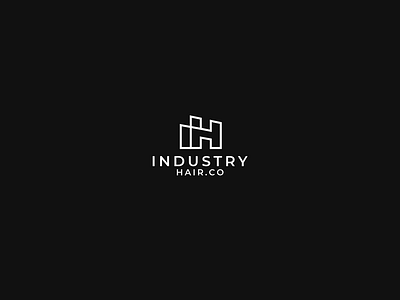The image showcases a simple, monochromatic design featuring a company logo on a solid black background. In the center, the white text reads "INDUSTRY" in all capital letters, with "HAIR.CO" positioned directly below it in smaller uppercase letters. Above the text, there is a minimalist line drawing constructed from white lines, forming a unique symbol that combines an 'H' and a stylized lowercase 'i' without the dot. The 'i' is slanted and integrates with the 'H', with the top line of the 'i' intersecting the middle of the 'H' and continuing to form its top section, while the bottom of the 'i' connects to the lower part of the 'H'. The entire logo and text are rendered in white against the black background, creating a stark, modern contrast with no additional colors or details present. This elegant, straightforward design is likely intended for web or print use, such as on a brochure or a company website.